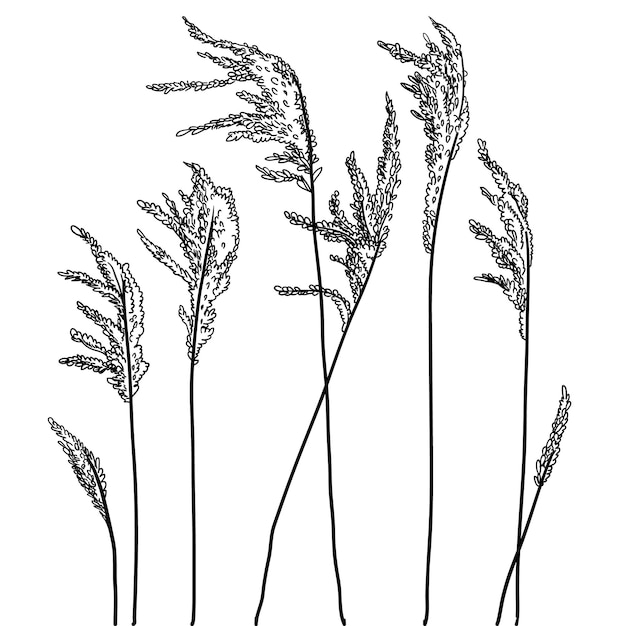This is a detailed black and white sketch of a series of eight plant stems, likely resembling wheat. The drawing has no border or text and is set against a stark white background. Each stem varies in height, with the shortest ones positioned on either end and the tallest in the center. 

Starting from the left, the first stem is thin with a teardrop-shaped leaf and minimal detail. The second stem is about twice the height of the first, and features more leaves or protrusions. The third stem is taller yet, with additional thin projections and a slightly flatter shape. The fourth, fifth, and sixth stems reach the maximum height, with the fourth one bending and crossing over the fifth, creating an X shape. Similarly, the seventh stem, which bends to the right, is shorter, matching the first stem's size and also forms an X with the eighth stem, which is tall and straight like the third stem.

The stems appear smooth and wiry, some leaning forward while others are bending backward, giving the impression of movement as if swaying in the wind. Despite the intricate leaf and stem details, the sketch maintains a monochromatic palette, reinforcing its simplicity and elegance. The artist has chosen not to include a signature, leaving the focus solely on the delicate interplay of the plant's forms against the unblemished white background.